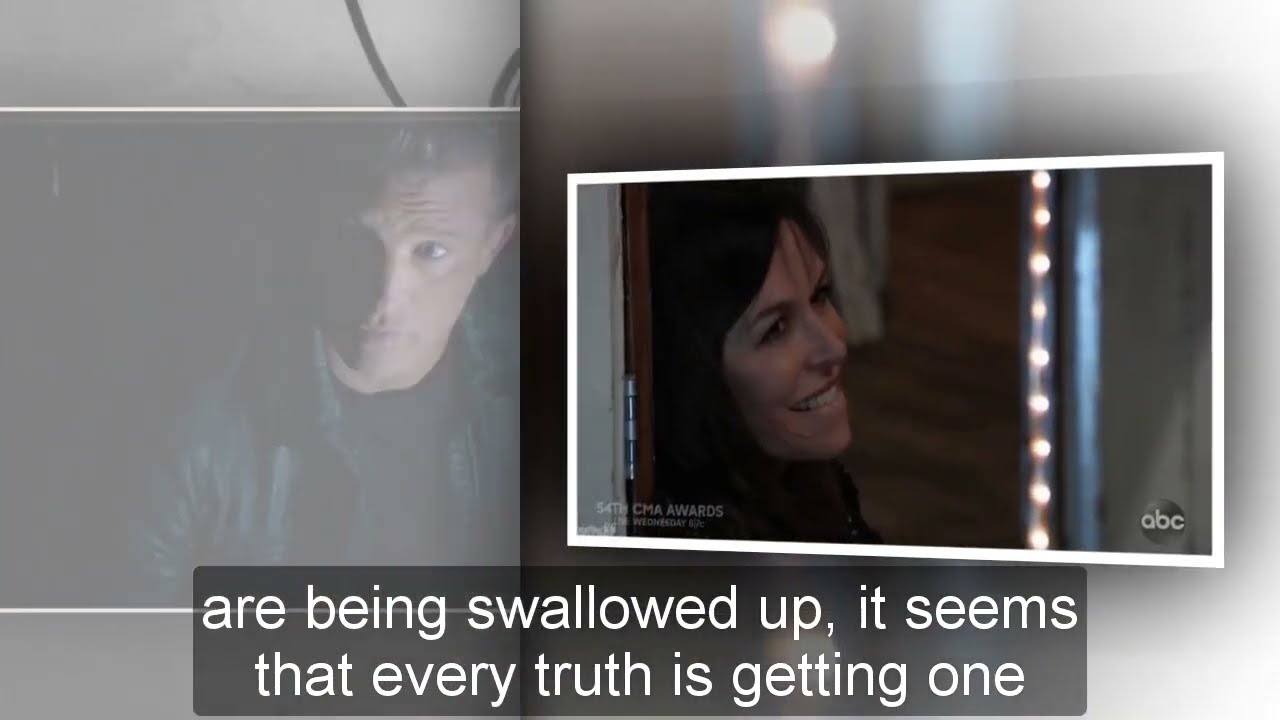The image is divided into two sections by a vertical line, both with a gray background and an abstract design. On the right side, there is a more focused photograph of a woman with dark, shoulder-length hair leaning against a doorframe. She has a straight nose, and wispy bangs, and is smiling warmly, looking slightly to her right. She is in an indoor environment with a wooden floor and various lights along the wall. In the lower right corner of her section, there's a circular disc with the ABC logo along with the text "54th CMA Awards".

On the left side of the screen, there is a faded photo of a man in a dark jacket. He appears to be in his late 40s or early 50s, with gray hair, and is of Caucasian descent. He is looking intensely to his left, slightly downwards, and his mouth is closed. The image captures only half of his face as he is turned away from the camera.

At the bottom edge of the overall image, in white letters on a gray block background, the text reads: "are being swallowed up, it seems that every truth is getting won."